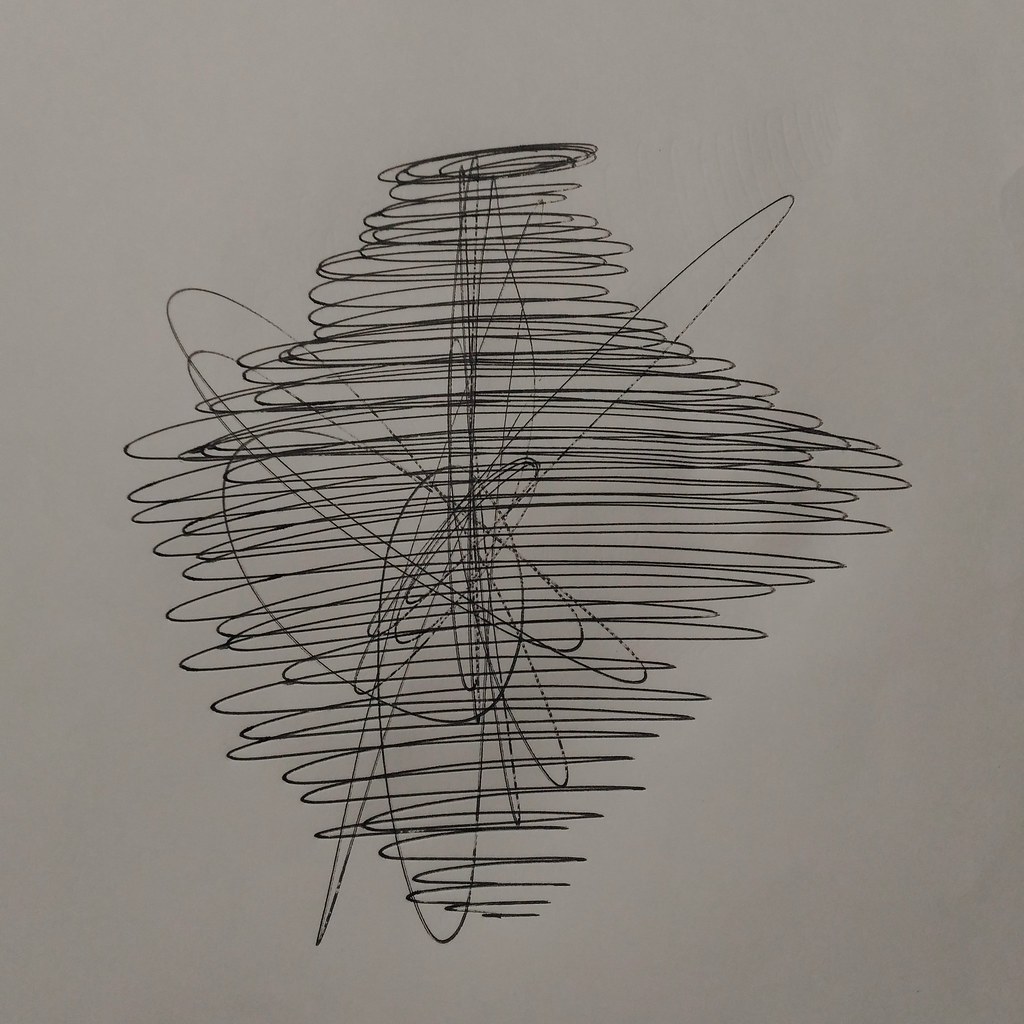The abstract artwork depicted features a predominantly dark gray background that varies in shade, becoming lighter in certain areas. Dominating the center of the piece are intricate black pen squiggles, forming an oval-like design. The composition starts with a lean, vertical arrangement at the top, expands into a wider section at the center, and tapers back to a lean, vertical pattern toward the bottom. These squiggles crisscross horizontally from left to right, creating a dynamic sense of movement. Additionally, there is a distinct X-shaped pattern formed by squiggles that intersect diagonally, spanning from the upper left to the lower right and upper right to lower left. The overall effect is a complex, textured interplay of black lines against the varying tones of the gray background, making a captivating and intricate abstract visual.